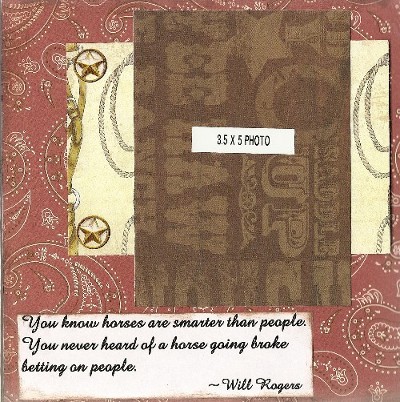The image displays various 3x5 and 3.5x5 photo papers with unique designs and semi-old appearances, characterized by different shades of brown and blurriness. One style features a cream background with tarnished gold etching. Overlaying these papers is a red paisley-patterned background resembling an old-time bandana with silver or white detailing. At the bottom left-hand corner of the image, there is a handwritten quote by Will Rogers, stating, "You know horses are smarter than people. You never heard of a horse going broke betting on people." Prominent in the design are layers including a dark pink mauve square with a white paisley design, a beige layer with gold stars and silver looping lines, and a brown rectangle with beige designs. A central white bar reads "3.5 by 5 photo" in black text, enhancing the layered and textured aesthetic.